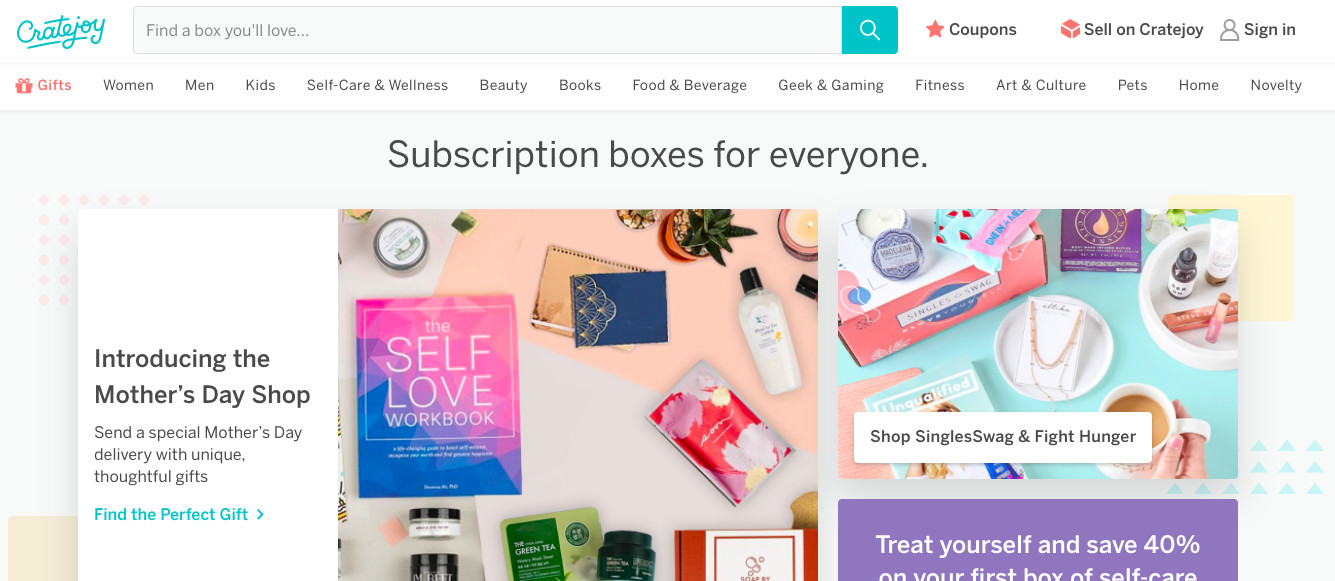The image is a promotional homepage for the website "Cratejoy." The website name "Cratejoy" is written in elegant blue cursive on a white background at the top. Below, a tagline reads, "Find a box you'll love," which is followed by a search bar that features a white find icon on a blue background.

On the right side of the page, there is a prominent red star with the label "Coupons." Next to it is a section labeled "Sell on Cratejoy" and options to "Sign In." Beneath this, the navigation menu offers various categories: "Gifts" in red, with other categories in black including "Women," "Men," "Kids," "Self-Care and Wellness," "Beauty," "Books," "Food & Beverage," "Geek & Gaming," "Fitness," "Art & Culture," "Pets," "Home," and "Novelty."

Below the navigation menu, a banner states "Subscription Boxes for Everyone" in black text on a white background. 

On the left side, there's a vertical white rectangle featuring a message about a special sale: "Introducing the Mother's Day shop. Send a special Mother's Day delivery with unique, thoughtful gifts." A blue button below this reads, "Find the perfect gift," accompanied by a right arrow.

Next to this is an image highlighting Mother's Day gift options including a "Self-Love Workbook," lotions, and various spa products such as face creams. Another image next to it promotes "Singles Swag," encouraging users to "Treat yourself and save 40% on your first box of self-care." The promotion includes items like a necklace, a cup of coffee, and incense.